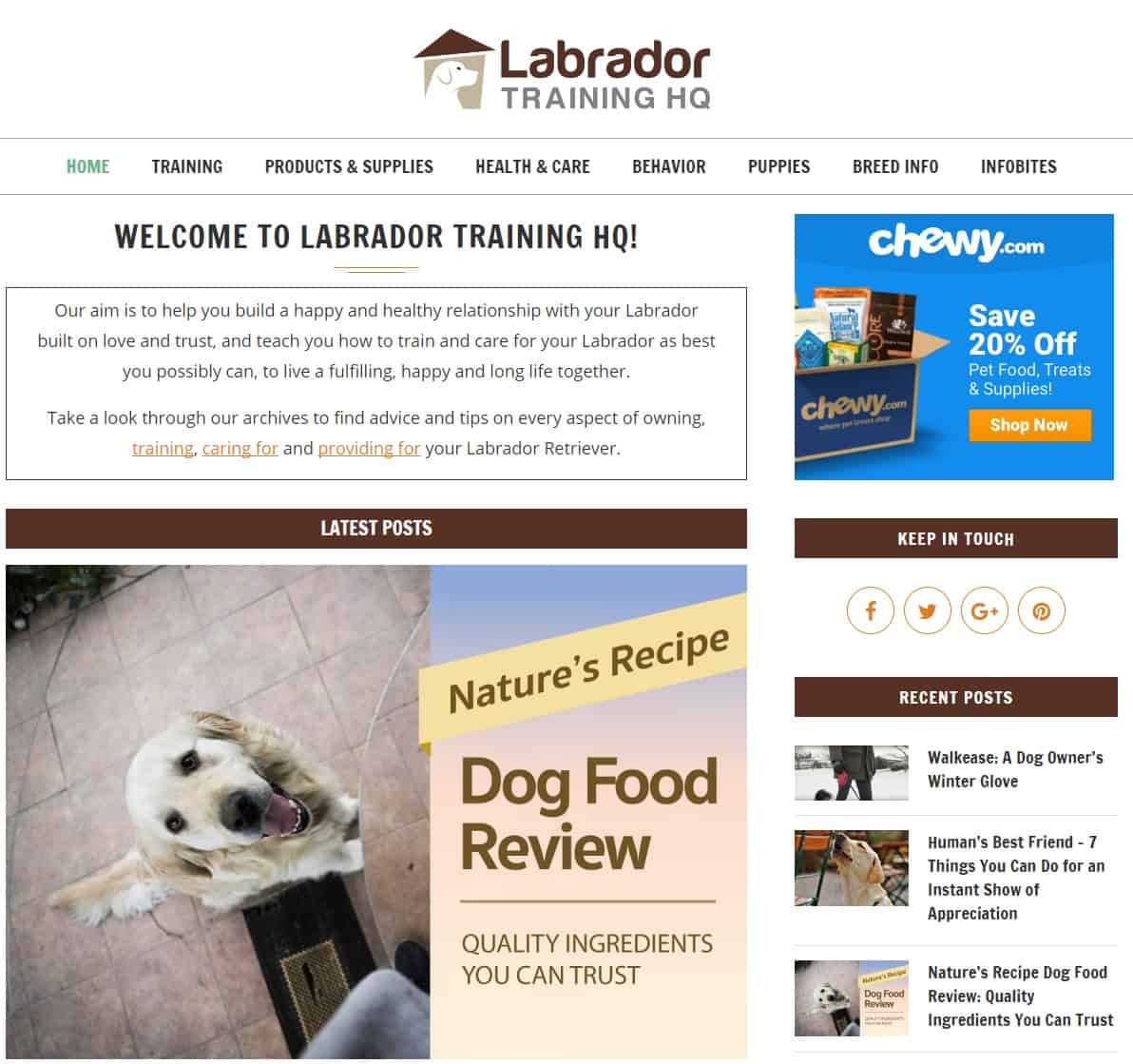The webpage titled "Labrador Training HQ" is dedicated to dog training, specifically focusing on Labrador Retrievers. The logo features a freehand, four-sided light gray shape, resembling a non-uniform quadrilateral, with a dog's profile silhouette within it. Topping the logo is a dark brown triangular roof, intentionally skewed to one side, giving it a whimsical touch. 

Beneath the logo lies the main menu, which includes tabs for Home (highlighted in green), Training, Products and Supplies, Health and Care, Behavior, Puppies, Breed Info, and InfoBytes. Directly under this menu, the welcome message invites visitors to explore content designed to help them build a healthy, loving relationship with their Labradors, anchored by trust and effective training. It encourages readers to browse through the archives for advice and tips on all aspects of Labrador ownership, from training and caring to providing for their pets.

Further down the page, the "Latest Posts" section features a photograph taken from above of a happy dog looking up and smiling. Adjacent to this image is a featured post titled "Nature's Recipe Dog Food Review: Quality Ingredients You Can Trust," which appears to be an advertisement.

On the right-hand side panel, there is an advertisement for Chewy.com, encouraging users to save 20% by shopping now. Below this ad, there are social media icons linking to the site's Facebook, Twitter, Google Plus, and Pinterest pages. Additionally, the "Recent Posts" section highlights three articles: "Walkies: Human's Best Friend," "Nature's Recipe Dog Food Review," and another, each accompanied by small thumbnail images.